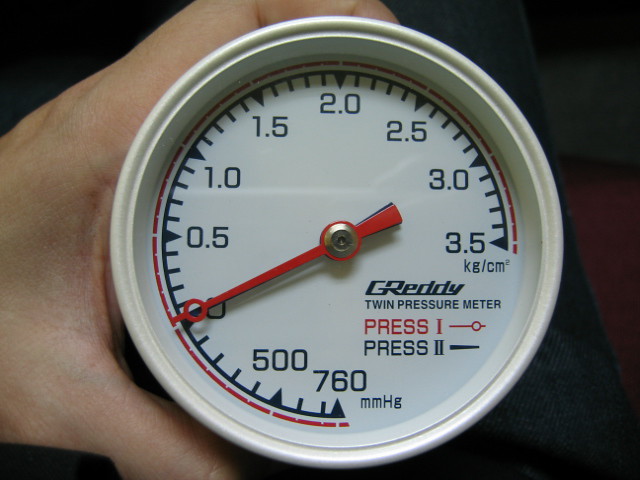A person is holding a G-Ready twin pressure meter, prominently displaying intricate details and craftsmanship. The meter's dials and face exude a sophisticated aesthetic, blending functionality with style. The right-hand dial indicates a pressure rating from 3.5 to 760 mmHg (millimeters of mercury), with precise graduations for accurate readings. The dial is adorned in vibrant red, while the meter's face and casing are a pristine white. The text and numbers are elegantly printed in navy blue, accented by subtle touches of red. The design around the numbers features a distinctive dark blue and red border, adding a layer of visual interest. The meter's appearance suggests it is well-suited for underwater activities, given its detailed and robust construction. The person's hand, partially visible, delicately grips the device, with a slight bend in the finger at the top and a glimpse of the thumb at the bottom, adding a human element to this technical instrument.